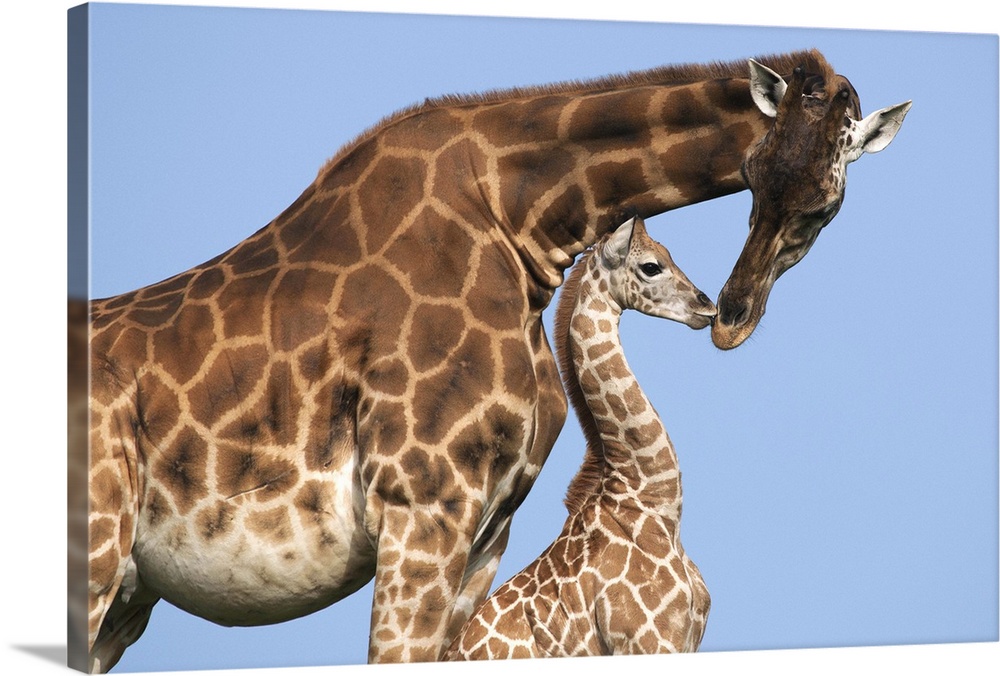This professionally taken photograph captures a tender moment of bonding between a mother giraffe and her baby. The scene is set against a vibrant, completely blue sky, enhancing the serene atmosphere. Both giraffes exhibit a captivating blend of neutral colors and distinctive patterns. The mother giraffe, with her dark brown fur and geometrical striped spots, has a white belly and a line of fur running down the back of her neck. Her black eyes and white ears add to her striking appearance. The baby giraffe, mirroring the mother's coloration but in a younger, smaller form, shares the same black eyes and white ears. Both giraffes are nuzzling each other, displaying an affectionate connection. The light blue background extends to the sides and underneath, creating a 3D effect. The image, appearing almost like it is on a canvas, suggests a deliberate artistic presentation, underscored by a subtle triangle shadow on the bottom left corner of the frame. This picturesque portrayal highlights the gentle interaction between the two animals, capturing a beautifully intimate moment in their natural habitat.